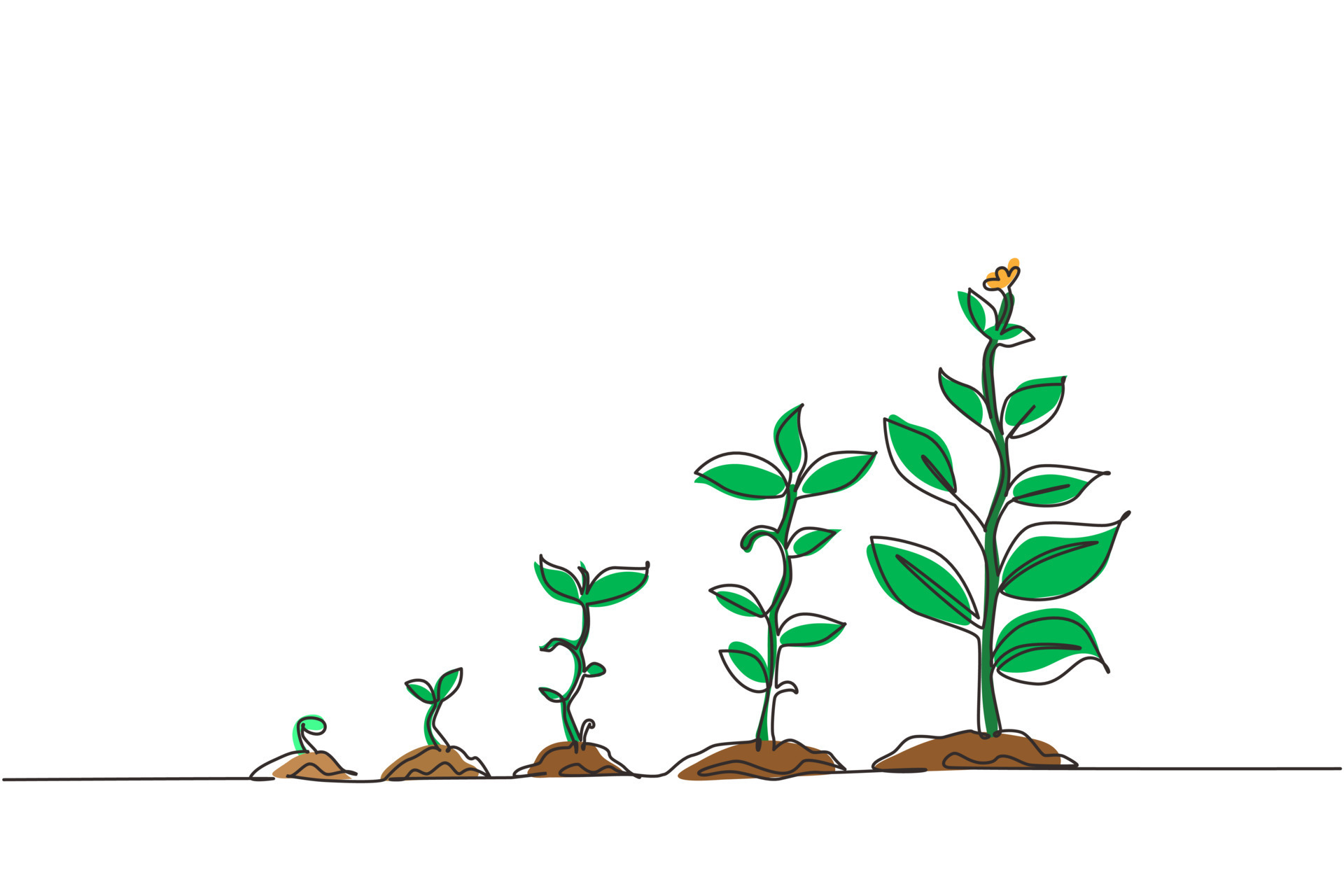This detailed illustration on a white background depicts the progressive growth of a flower at five distinct stages, delineated along a black line. The art style is sketch-like, with a color palette limited to black, brown, green, and yellow. On the far left, a small mound of brown soil nurtures a nascent light green sprout. Moving rightward, the second stage reveals a slightly larger sprout with two budding leaves. The third stage shows further growth, with the two initial leaves becoming more prominent and additional leaves beginning to form. By the fourth stage, the plant is taller with fully expanded leaves, robustly reaching toward the light. In the final stage, the plant stands the tallest, adorned with large, mature leaves and a budding yellow flower at the apex, poised to bloom.